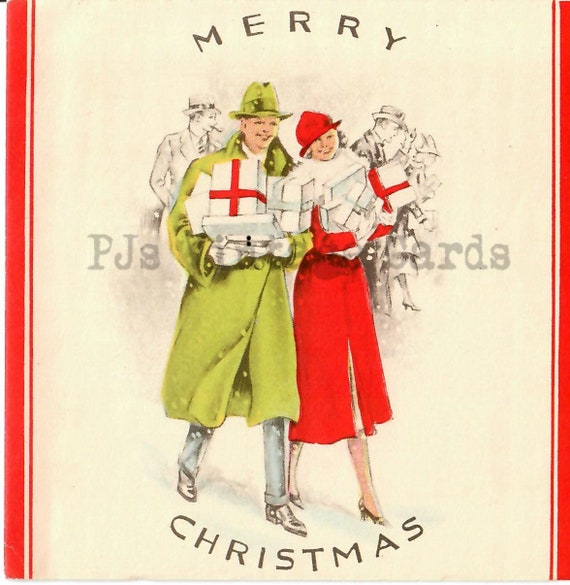This nostalgic, hand-drawn Christmas greeting card from PJ's Cards features a cheerful couple in the foreground, vividly brought to life with pops of color against a cream background. The card is bordered with red trimmings, and at the top, it reads "Merry" in arched block letters, mirrored with "Christmas" at the bottom. The gentleman, adorned in an olive green coat with a matching hat, carries an array of gifts wrapped in white boxes with red and silver ribbons. Beside him, a lady in a knee-length red coat and matching red hat also carries several presents, her face lit up with a smile. The background features black-and-white sketches of people dressed in suits and hats, adding a nostalgic feel to the festive scene.